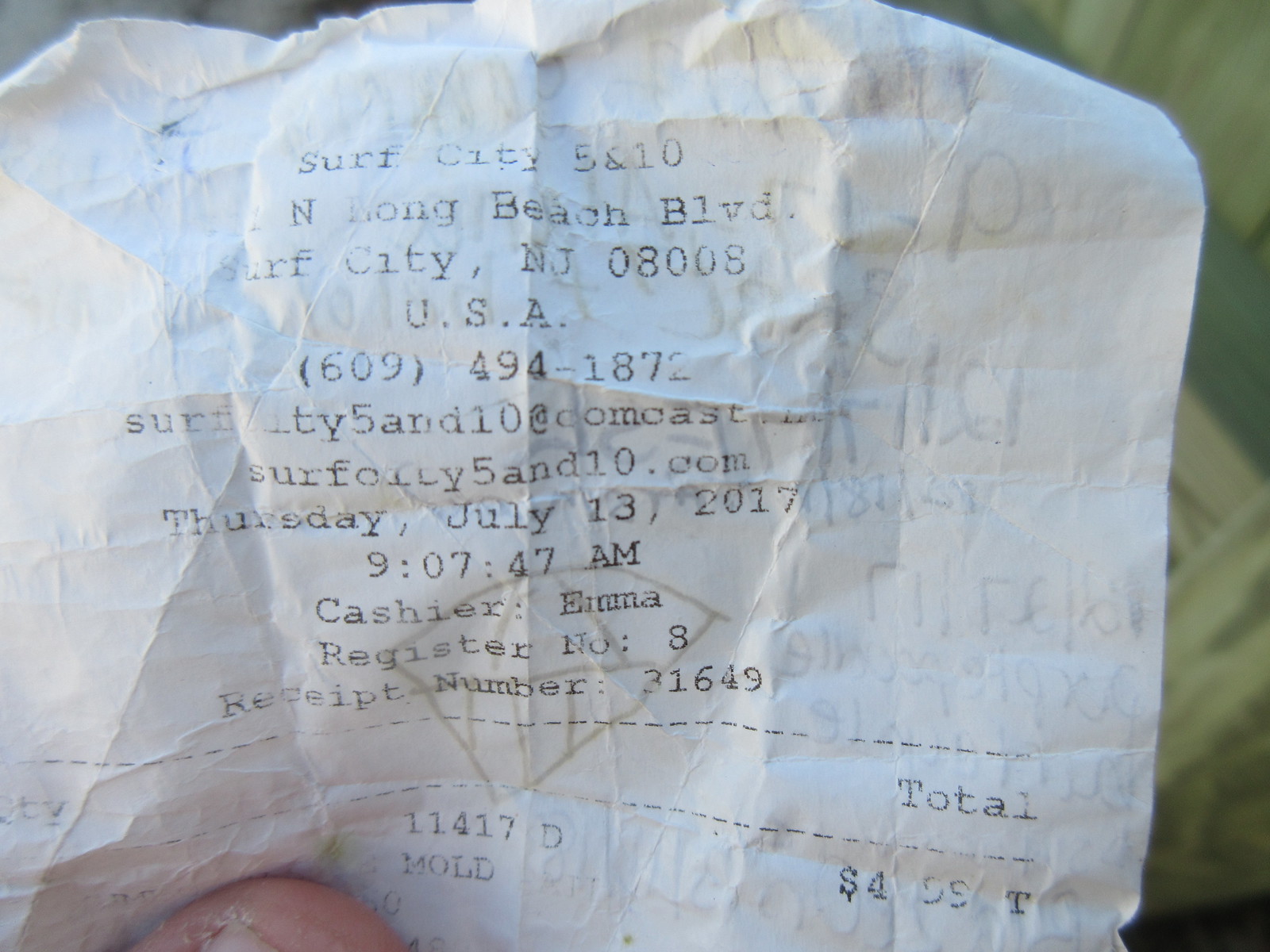This is a close-up photo of a worn-out, slightly faded receipt from Surf City 5 and 10, located at North Long Beach Boulevard, Surf City, New Jersey 08008, USA. The top of the receipt includes the store's phone number: (609) 494-1872. The receipt also lists the website, although parts of it are illegible, suggesting something like 'surfcity5and10.com' or 'surffolly5and10.com'. The transaction took place on Thursday, July 13, 2017, at 9:07 a.m. The cashier was Emma and the transaction was processed at register number 8. The receipt number is 31649, with a total purchase amount of $4.99, noted with a 'T' next to it. The left side of the receipt displays the word 'quantity' but the number is not visible. Below the total is the code 11417D, followed by the term "MOLD." A corner of someone’s thumb is holding the receipt, adding a personal touch to the image. Additionally, there are faint pencil markings that seem to have been erased, further contributing to the worn appearance of the receipt.